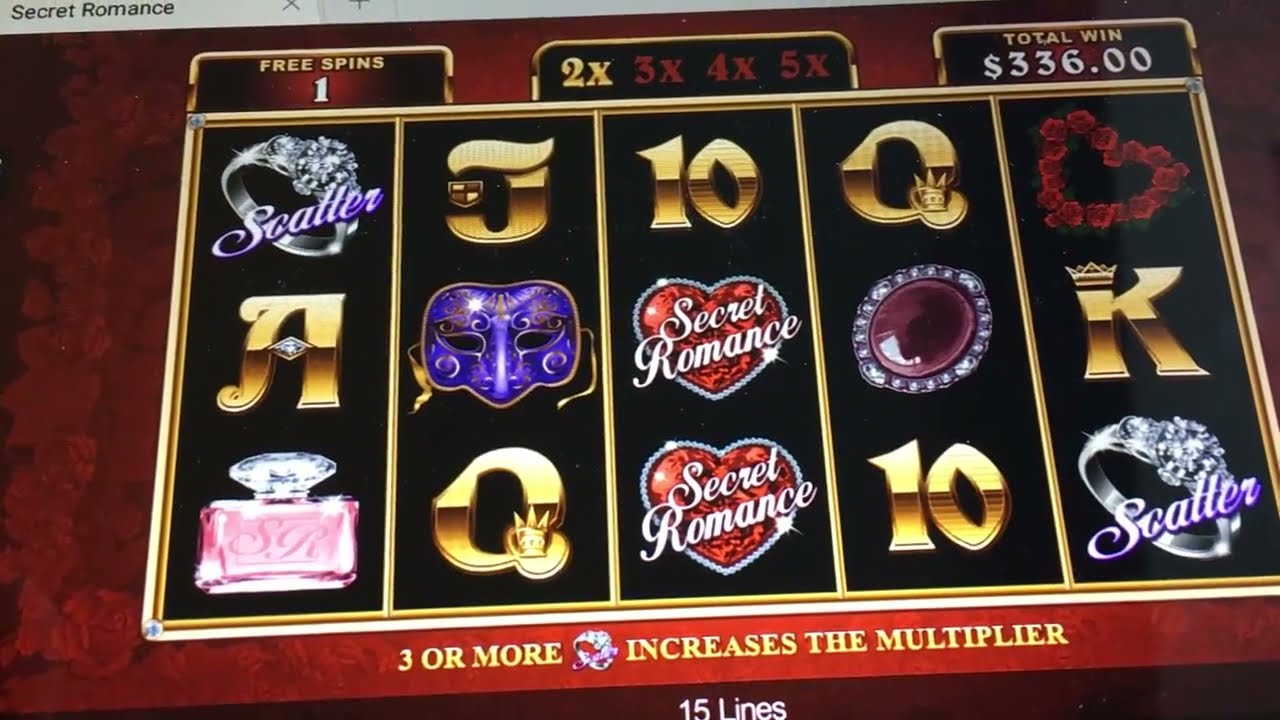The image captures the Secret Romance slot machine on a website, viewed within a browser window. The browser tab in the top left corner labeled "Secret Romance" signifies this. The slot machine's interface dominates the screen, characterized by five vertical columns filled with symbols that include letters, numbers, a diamond ring, a perfume bottle, heart shapes, a mask, and a brooch. Above these columns, the text displays “Free Spin 1,” and a multiplier grid ranging from "2x" to "5x" in gold and maroon fonts. The total winnings amount to $336.00, presented in white font. Additionally, instructions state that "3 or more increases the multiplier," highlighting the game’s rule where obtaining three or more diamond rings marked "Scatter" boosts the multiplier. The game operates across 15 lines, with a striking red background adorned with elegant designs.